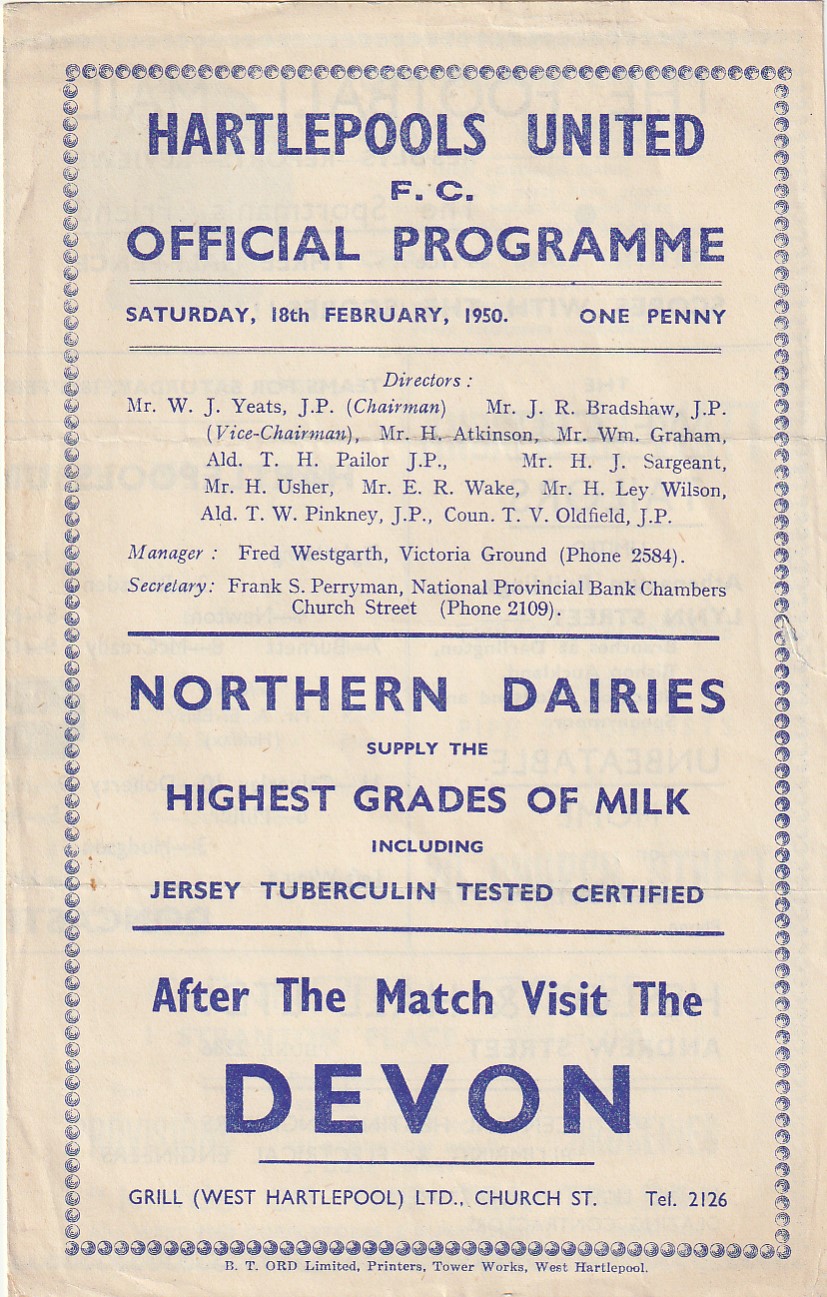This image displays a vintage, tan-colored program cover for Hartlepool United FC, dated Saturday, 18th February 1951, priced at one penny. The page features an intricate blue border made of small soccer ball illustrations. The program title, "Hartlepool's United FC Official Program," is prominently printed in bold black text at the top. Below the title, there's detailed text listing club officials: Chairman Mr. W. J. Yeats, Vice Chairman Mr. J. R. Bradshaw, along with directors including Mr. H. Atkinson, Mr. William Graham, Mr. T. H. Paler, and others. Key management personnel like Manager Fred Westgarth (located at Victoria Ground, phone 2584) and Secretary Frank S. Perryman (National Provincial Bank Chambers, Church Street, phone 2109) are also mentioned. Following this text, an advertisement for Northern Dairies highlights their high-quality, certified milk, including Jersey Tuberculin tested milk. A subsequent line invites readers to visit the Devon Grill in West Hartlepool after the match. At the very bottom, the page includes the printer's information: "B.T. Ord Limited, printers, Tower Works, West Hartlepool." The overall presentation of the program effectively captures the essence of a mid-20th century football club's match-day material.